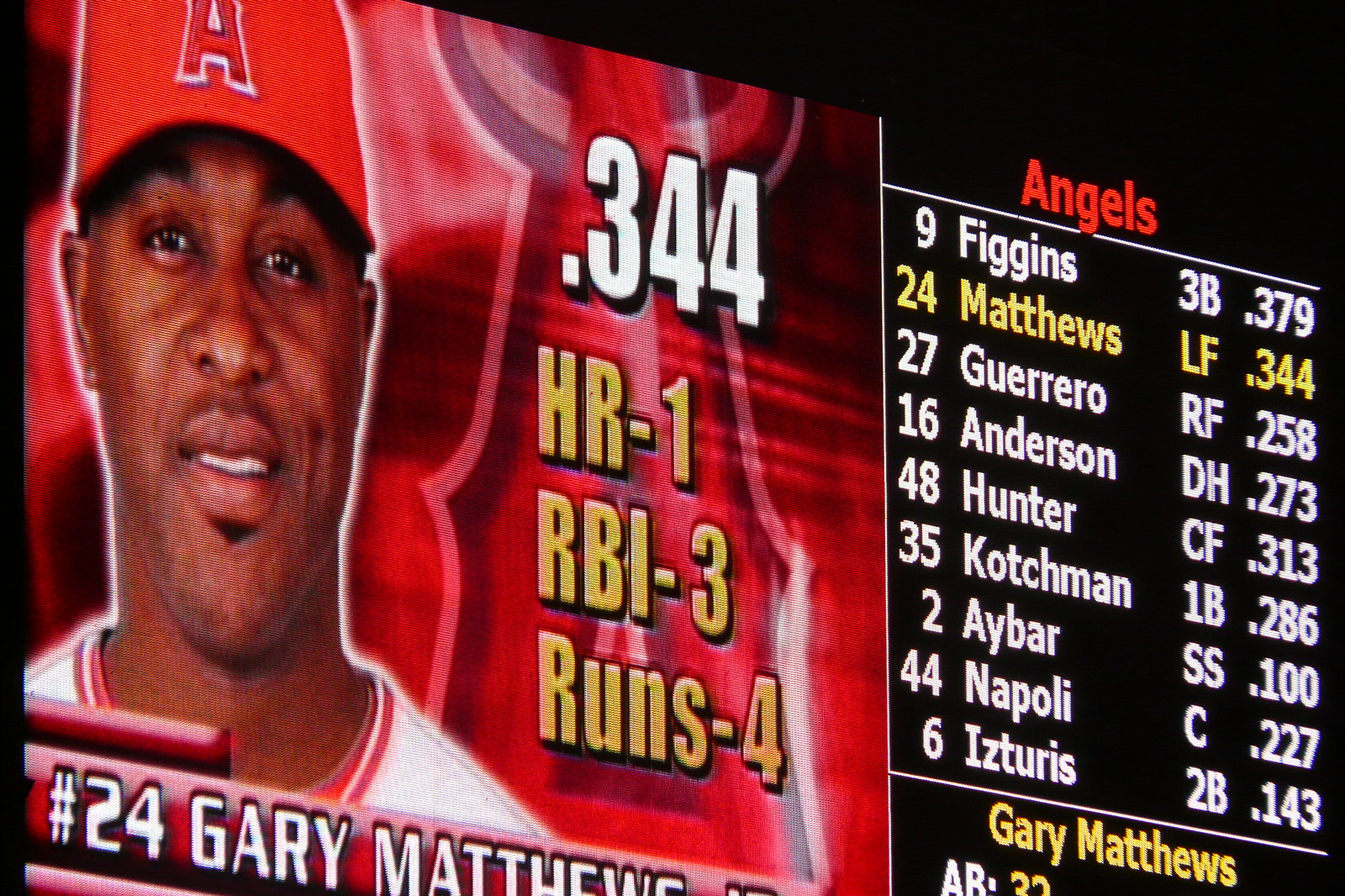This image features a detailed digital scoreboard set against a black background. On the left side of the scoreboard, there is a photograph of a black player, Gary Matthews, who is wearing a red baseball cap with a white letter 'A' on it, indicating he plays for the Angels. He is dressed in a white and red uniform. Displayed next to his image are his statistics: a batting average of .344, 1 home run (HR), 3 runs batted in (RBI), and 4 runs. The main part of the scoreboard lists the team's name in red, "Angels," followed by the lineup and their statistics, including:

1. Figgins, 3B - .379
2. Matthews, LF - .344
3. Guerrero, RF - .258 (or 'Gooderot' as some transcriptions suggest)
4. Henderson, DH - .273
5. Hunter, CF - .313
6. Coachman, 1B - .286
7. Ibar, SS - .100 (likely a misspelling of "Ivar")
8. Napoli, C - .227
9. Histories, 2B - .143 (possibly a mishearing, but meant to be "Deserters")

Gary Matthews' name is repeated below the scorecard, along with additional text and numerical information: "AB.32".